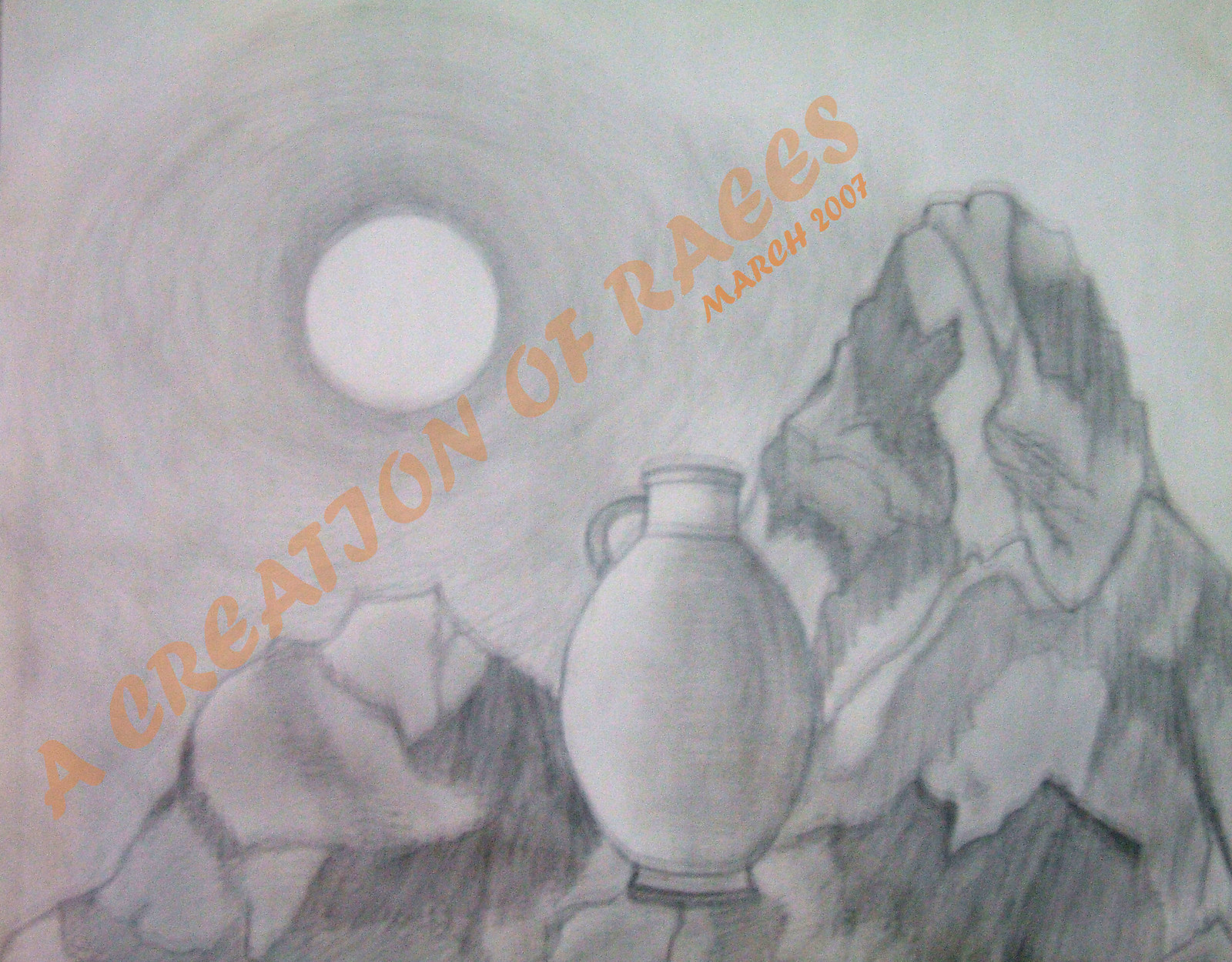A meticulously sketched image rendered in a spectrum of white, gray, dark gray, and charcoal hues. Dominating the bottom right side of the composition is a heavily shadowed rock or mountain range, which peaks prominently on the right and slopes gently downwards toward the lower left corner. Intricate and varied shading techniques give this rock a textured, almost tactile appearance. Nestled in the center of the rock is a white urn, accentuated with subtle gray shading. The urn features a conspicuous handle near its top, positioned on the left side. The upper left corner of the piece showcases a white sky, interspersed with shades of sketched gray, creating a sense of depth. Prominently featured is a large white area symbolizing the sun, from which pale gray, ring-like lines radiate outward. Diagonally bridging the space between the sun and the mountain, light orange lettering spells out, "A creation of rays," followed by "R-A-E-E-S." The artist's signature is also present, though it is too small to be deciphered.